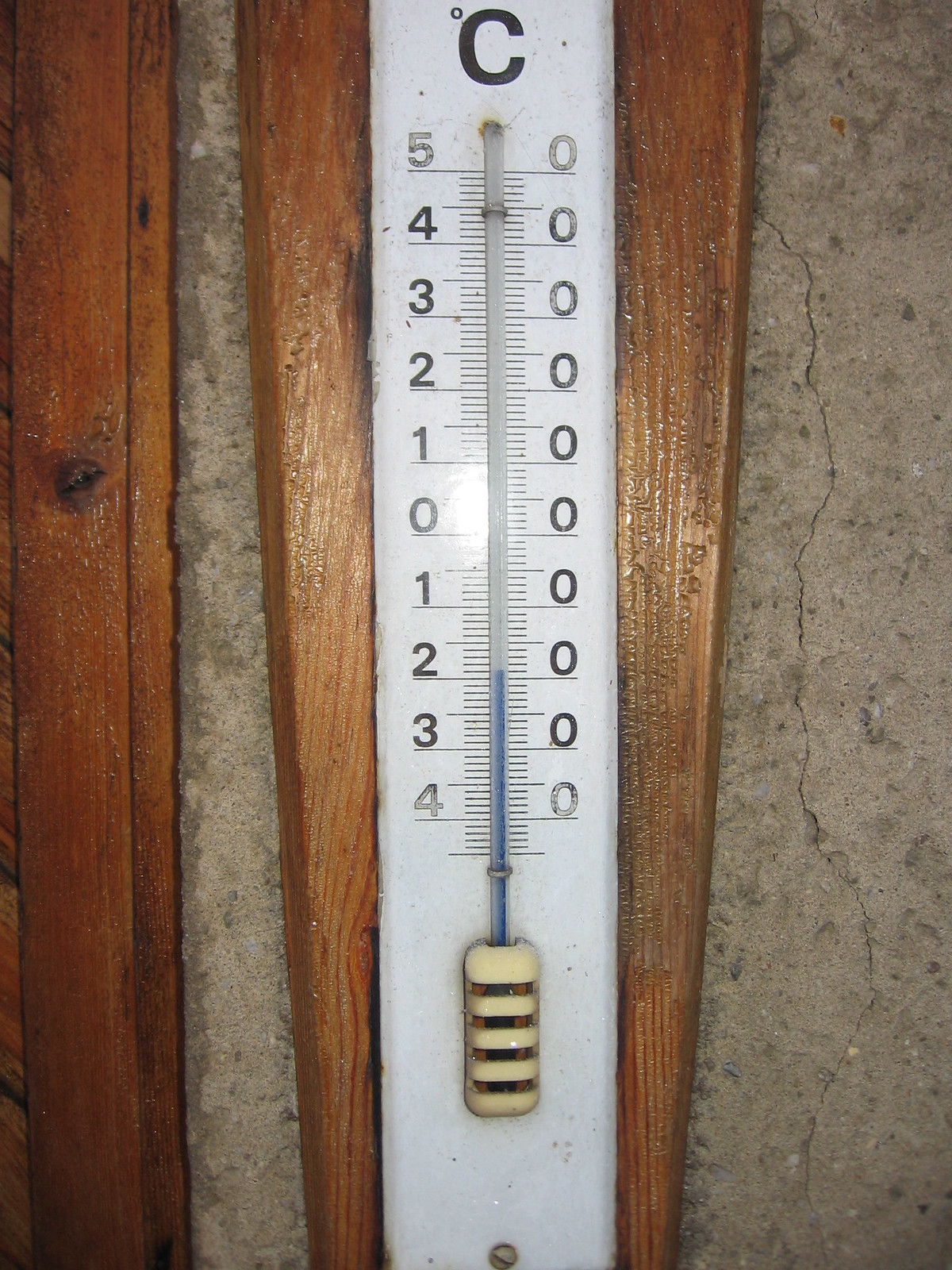In this vertically-oriented color image, a white thermometer is prominently displayed. The thermometer features a thin mercury tube running vertically through its center, positioned atop a sleek white metal plate. On either side of the tube, black numerical markings are clearly visible, detailing temperatures in degrees Celsius. The liquid inside the tube appears as a dark blue, adding contrast to the white backdrop. At the top of the tube, a bold "C" denotes the temperature scale. The temperature readings on the left side of the plate ascend from 5 down to 0, and then continue from 1 down to 4 in a vertical sequence below the 0 mark. Meanwhile, all numerical values on the right side of the tube are 0s. Regularly spaced hash marks along the tube provide precise measurement intervals.

The entire thermometer plate is mounted on a piece of wood, which is securely fixed to a plaster wall. The wall itself is visibly aged, adorned with noticeable cracks that hint at the passage of time. The overall composition of the image draws a stark contrast between the meticulously designed measuring instrument and the weathered, imperfect backdrop.